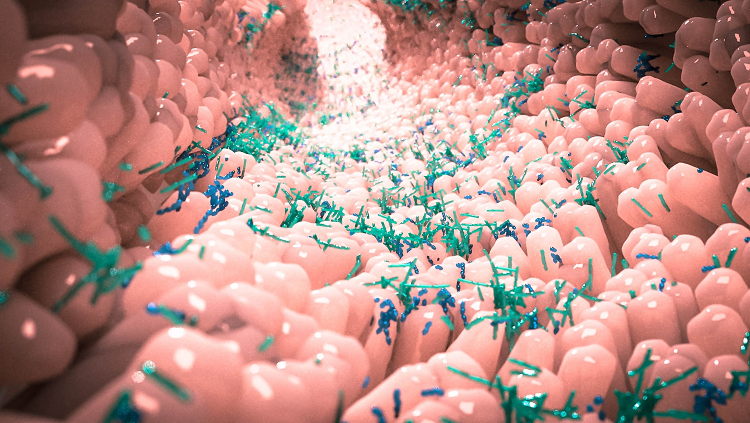The image depicts a computer-generated environment resembling the interior of a biological tube, possibly part of a digestive system or blood vessel. The tunnel walls are formed by numerous shiny, light pink cylindrical structures, reminiscent of the inside of a mouth but slightly lighter in color. These pink cylinders create a textured surface, protruding inward towards the tunnel's open space. The tunnel is illuminated by a light source extending from an unseen point, casting a gradient from light pink in the center to darker pink on the sides. Scattered throughout the tunnel are thin, sprinkle-like elements in shades of pine needle green and darker blue. These tubular fragments float freely, predominantly in the central space, adding a layer of complexity and color contrast to the scene.